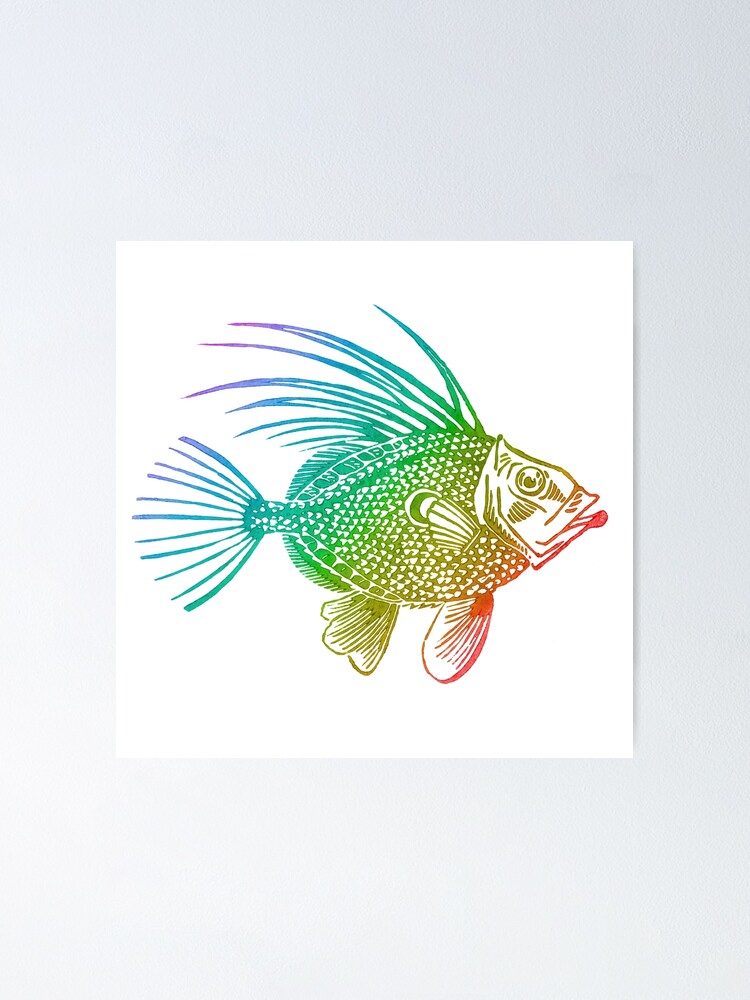This highly detailed, colorful drawing portrays a rainbow-colored fish on a large white piece of paper, set against a blue background. The fish, which appears flat and stamped with vibrant ink, faces to the right and boasts an array of colors that transition from red at the lips to blue and purple at the tail. The fish's body features a harmonious blend of light green, dark green, and red-orange scales. Its fins are distinctly spiky and elongated, with nine prominent ones on top in shades of purple, blue, and green, while the two underneath mix red and green hues. The fish’s mouth is slightly open, revealing its wide face, and its eye, open and attentive, looks directly at the viewer. Overall, the fish occupies a substantial portion of the paper, capturing attention with its striking, multi-colored appearance and intricate, dotted detailing.